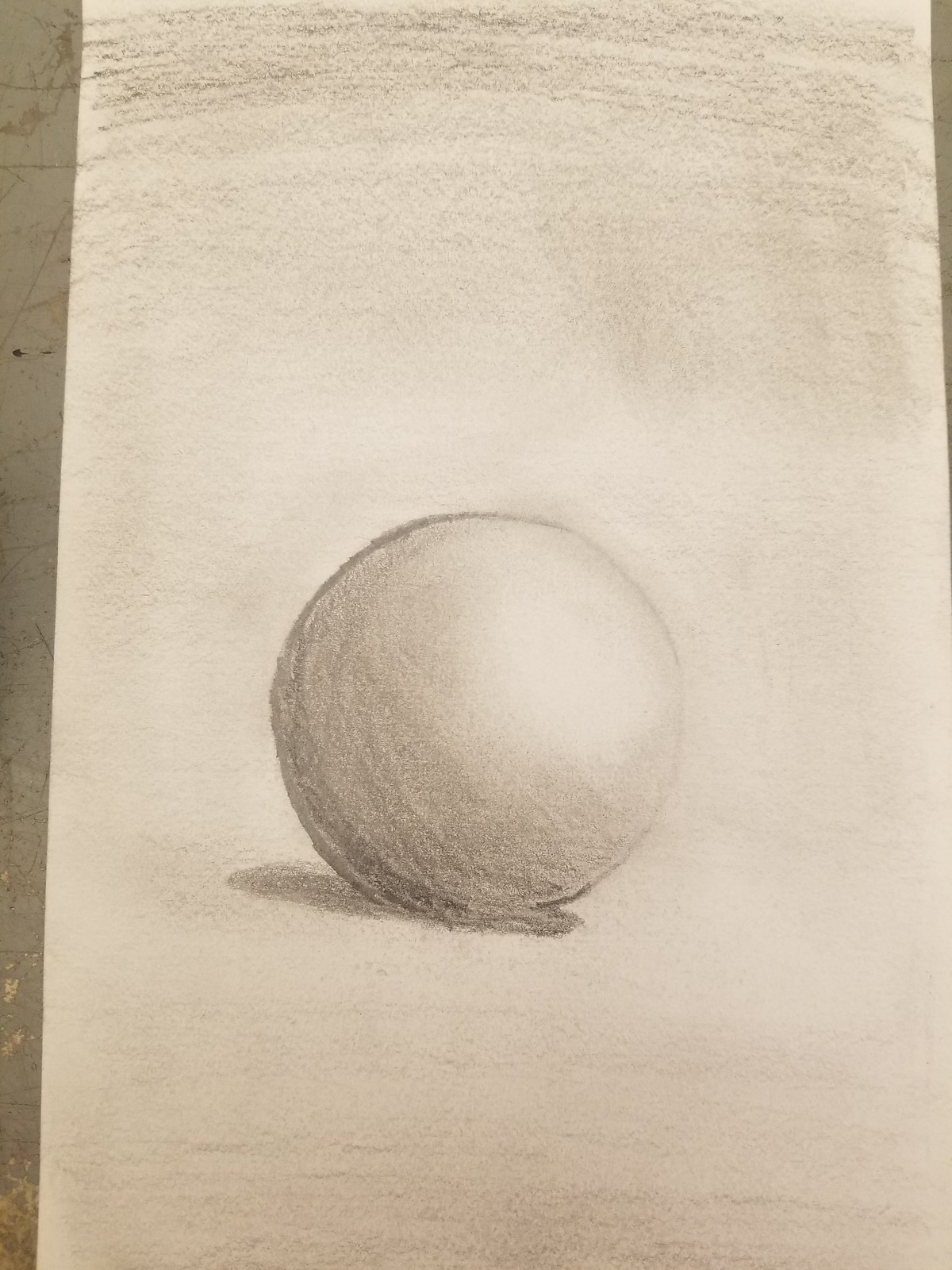A detailed and cleaned-up caption for the image could be:

"Resting on a pristine white marble countertop adorned with elegant gold streaks, a meticulously drawn pencil sketch captures the essence of a ball. The artwork, created on a crisp white sheet of paper, showcases a perfectly round circle, indicating the outline of a ball. The right side of the ball is gently highlighted, while the left side and the area beneath the ball are skillfully shaded to create a sense of depth and dimension. The shading intensifies directly below the ball, blending into a softer shadow that extends slightly to the bottom left. The top of the ball features subtle, darker scribbles, adding texture and contrast to the otherwise smooth finish. The base of the ball's shadow also displays delicate scribbling, executed with the side of the pencil, enhancing the realism and three-dimensional effect of the drawing."